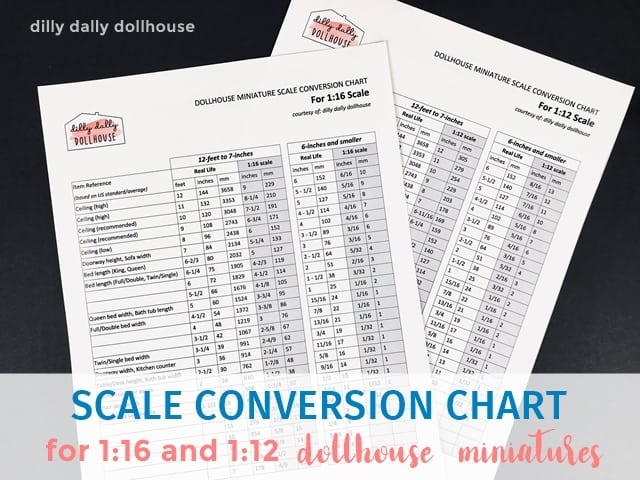This detailed image features a digitally synthesized photograph displaying two white papers with large, intricate charts on them containing columns of numbers and black writing. The prominent paper takes up a significant portion of the image, extending off the bottom edge, while the second paper is placed beneath it, more towards the right side. The top left-hand corner of the image features the text "Dilly Dally Dollhouse" in elegant black cursive, accentuated by artistic pink splatters and framed with a simple black house outline, resembling a logo. The charts are identified as "Dollhouse Miniature Scale Conversion Chart," with the first chart labeled "1:16 scale" and the second "1:12 scale," both in black text. Below these papers, a semi-transparent white or gray bar spans the bottom of the image, featuring the bold, blue capitalized text "SCALE CONVERSION CHART" and below, in smaller pink lettering, the specifics "1:16 and 1:12 Dollhouse miniatures," set against a plain flat black background. The conversion charts themselves are designed to help translate full-scale dimensions into miniature scales, containing numerous numbers to assist with the scale adjustments for dollhouse miniatures.